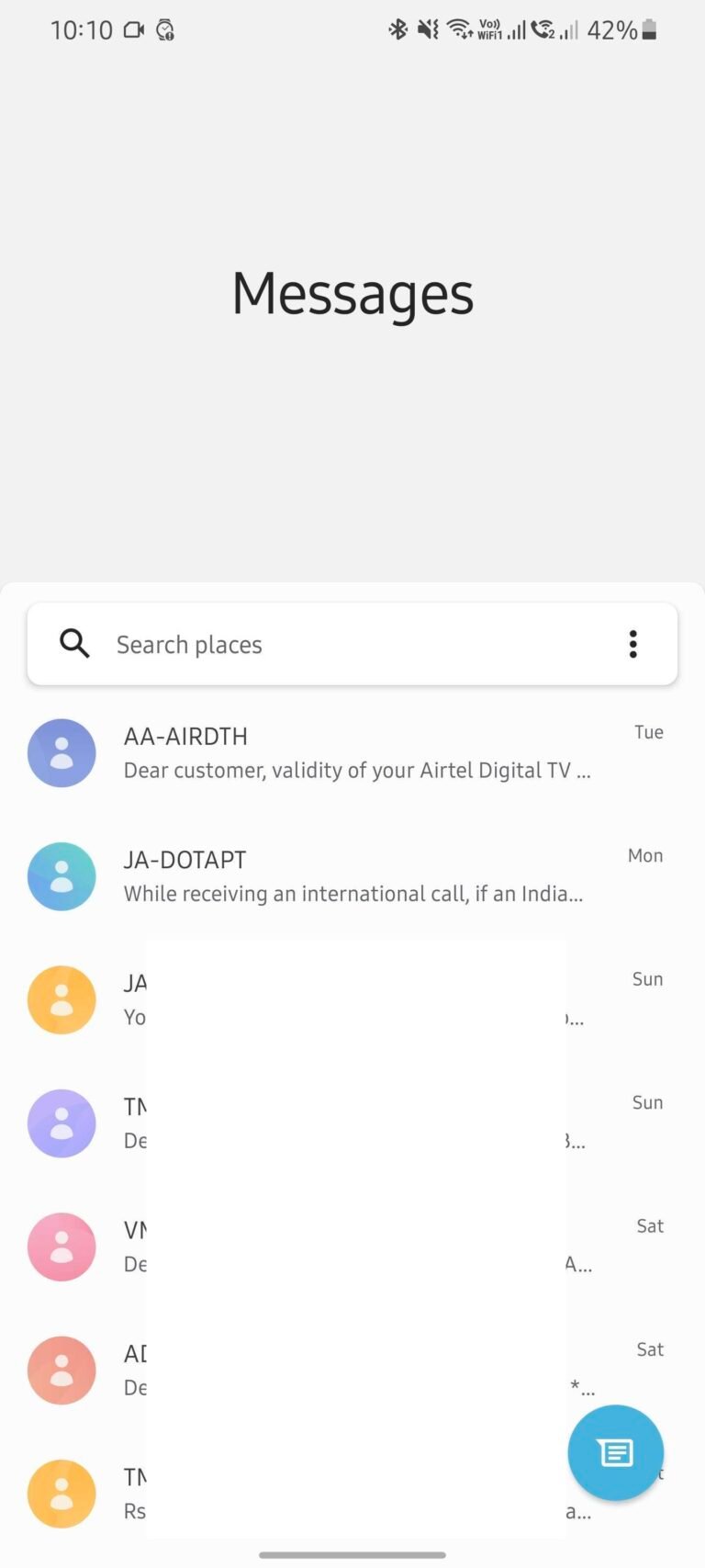A screenshot of a messaging app menu is displayed. At the top, the screen shows a header with the time "10:10" and several status icons: a camera icon, a circle icon, a Bluetooth symbol, a muted speaker icon, a Wi-Fi symbol, signal strength bars, a phone icon, and a battery indicator at 42%. Below this, a large gray box is labeled "Messages". 

Further down, there is a white search box with gray text and a black magnifying glass icon. The text reads "Search places" and is followed by three black dots.

Beneath the search bar, there is a series of colored circles, each containing an icon representing a person's head and shoulders. Next to these icons are brief snippets of messages:

1. A periwinkle circle labeled "AA AIR DTH" with the message fragment, "Dear customer, validity of your Airtel digital TV...". This message is dated "Tuesday TV".
2. A teal circle labeled "JA.apt" with the message starting, "While receiving an international call if an Indi...". The message is dated "Mun".
3. A gold circle showing "JA" and "YO" with the date "Sunday".
4. A lavender circle labeled "TM" with the message start, "DE...". The date is also "Sunday".
5. A pink circle starting with "VM" and the message part "DE...". The date here is "Saturday".
6. An orangey-pink circle with "AD" and the message part "DE...". The date is "Saturday".
7. Another gold circle showing "TMRS" with the start of a message.

Lastly, at the bottom of the screen, there is a blue circle with a white text bubble icon and a gray line separating the bottom section of the screen.